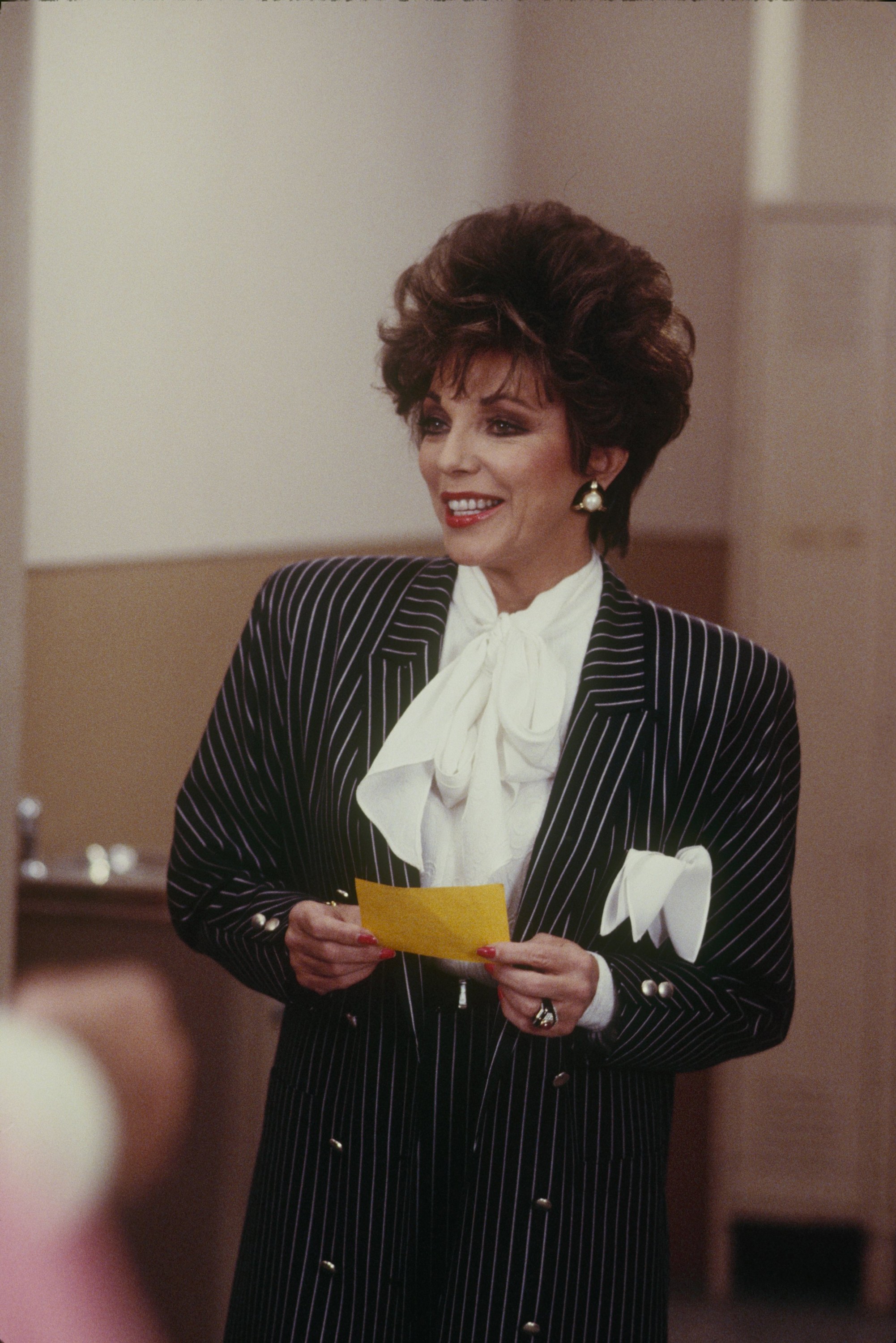The image is a color photograph from an old TV show, likely from the 60s or 70s, featuring a middle-aged woman standing indoors against a blurred, brightly-lit background with beige and white walls. The woman, who has lighter skin and short, poofy brown hair, is dressed in a black pinstripe business suit with a white undershirt and a flowy white scarf tied around her neck. She accessorizes with large earrings, red lipstick, red fingernail polish, and a large ring on her left ring finger. She stands centered in the image, visible from the waist up, holding a small yellow sheet of paper with both hands while smiling and looking towards the left, suggesting she is engaged in speaking or addressing an audience.